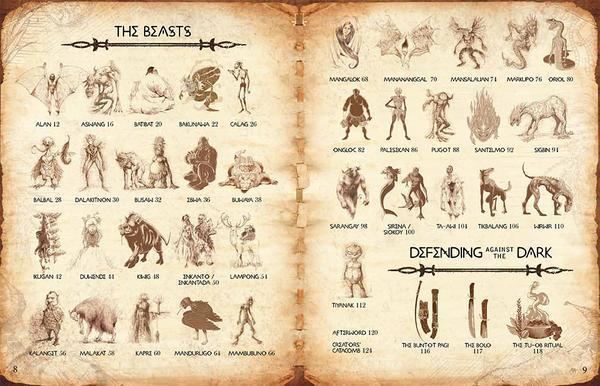This image captures an illustration, likely from an old book or perhaps a medieval-themed video game or comic book series. The pages appear worn and yellowed with simulated damage at the edges, giving them an ancient, aged look. On the left page, there is a heading in an old-looking font that reads "The Beasts." Below this heading, there is a spiky horizontal divider. The page is divided into four rows, each containing five columns of detailed illustrations, depicting twenty different beasts. Each beast is labeled with its name and accompanied by a number, possibly indicating a page number or a health rating. The beast names include Alan, Ashwing, Clag, and other less familiar ones, each illustrated in dark brown.

The right page continues this layout with three more rows of five beasts, followed by a single, standalone beast beneath these rows. In total, there are approximately twenty-five to thirty characters spread across both pages, showcasing a mix of medieval fantasy creatures such as half-man half-bat, half-rat, and a cat-like creature with hooves. The illustrations suggest a thematic context, possibly an in-game guide or a catalog of characters. In the lower right corner of the right page, the text "Defending Against the Dark" introduces a section that lists various weapons, each named and numbered, perhaps hinting at utility in either a game or a narrative context. The overall presentation suggests it serves as a table of contents or an in-game directive, neatly cataloging the beasts and weapons for players or readers.